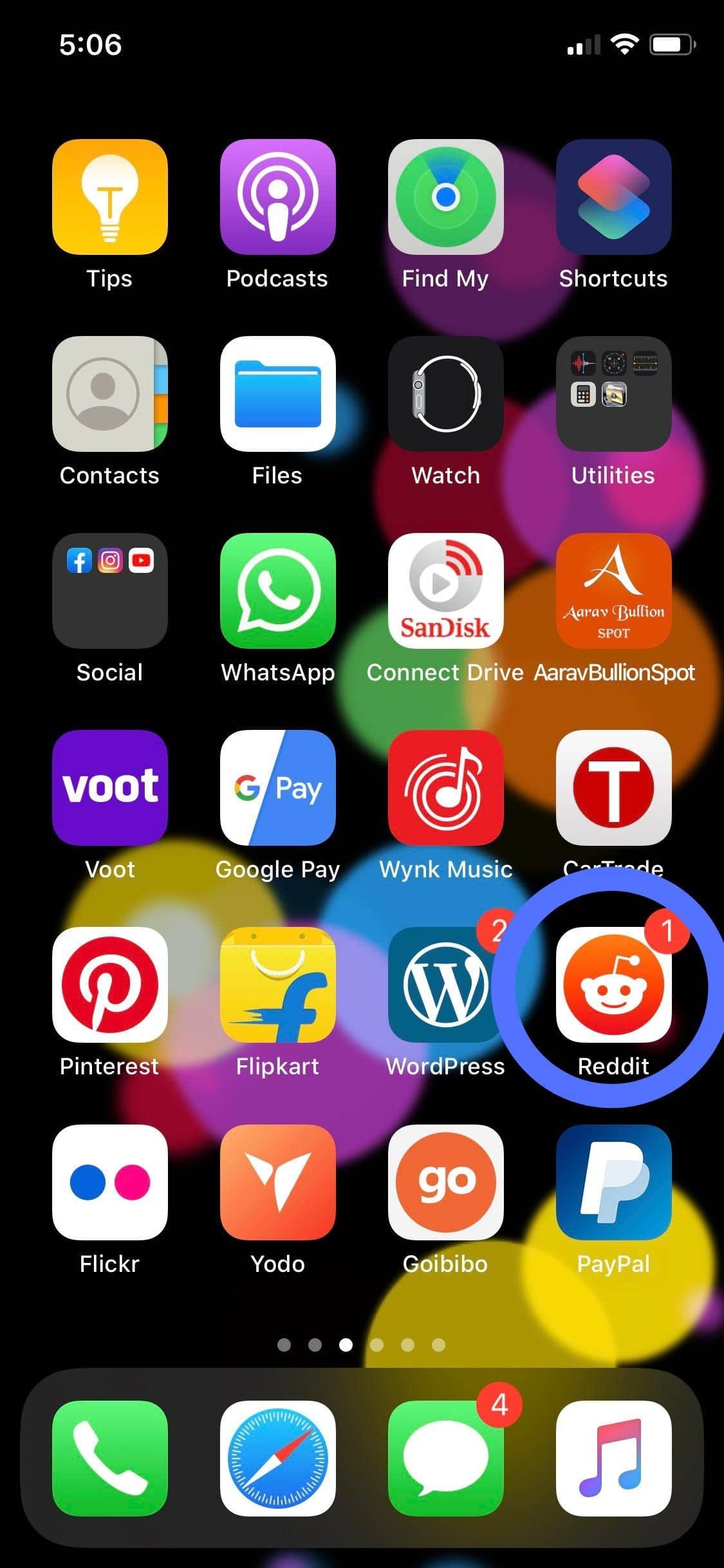The screenshot displays the homepage of a person's smartphone, captured at 5:06 PM. The top bar illustrates two bars of reception and a full Wi-Fi signal, alongside a predominantly full battery life indicator.

The layout consists of four columns and seven rows of app icons:

- **First Row:** Four app icons.
- **Second Row:** Four app icons.
- **Third Row:** Contains a folder labeled "Social" holding three social media apps, and an additional app (WhatsApp) next to it.
- **Fourth Row:** Four app icons.
- **Fifth Row:** Four app icons.
- **Sixth Row:** A highlighted app icon encircled in blue, specifically for Reddit.
- **Seventh Row:** Four apps, including Flickr, Yodo, Go, and PayPal.

Beneath the app grid, there are six dots, indicating the current page out of several app pages, with this particular screenshot showing the third page. At the very bottom, the dock contains four essential apps: the phone app, Safari browser, iMessage, and Apple Music.